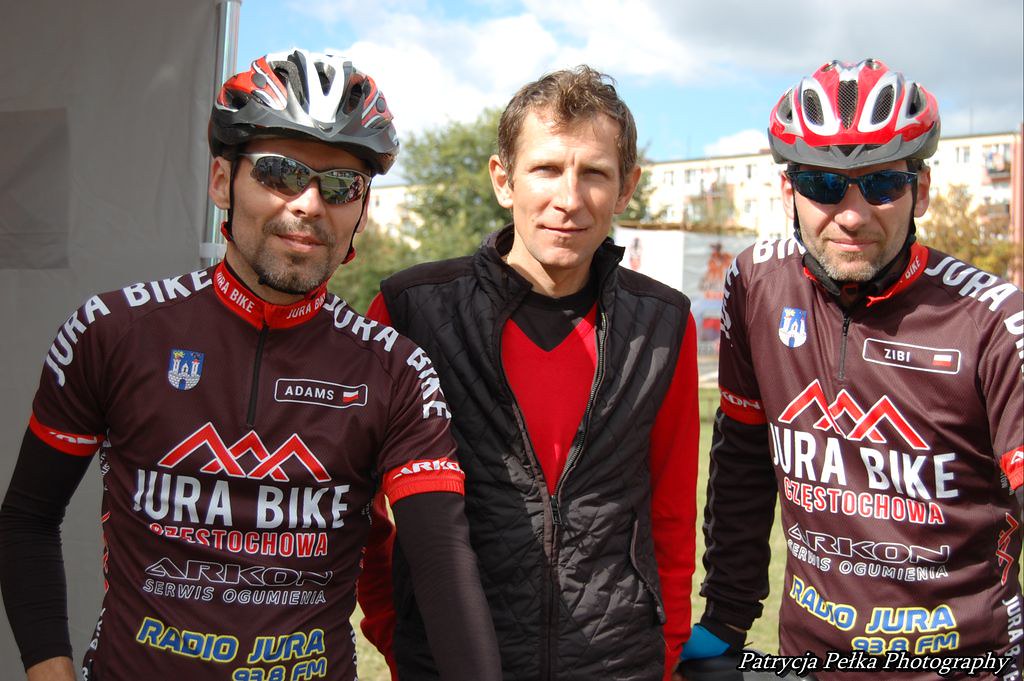In the vibrant full-color photograph, set against a backdrop of clear blue skies with scattered clouds, three men stand in front of indistinct buildings and trees. The man in the middle sports a white long-sleeve shirt paired with a gray sleeveless vest, along with short hair. Flanking him on both sides are two men clad in bike racing gear and helmets, each adorned with sunglasses.

The two cyclists, identified by name tags as Adams on the left and Zibi on the right, both have a few days' worth of beard growth. Their racing shirts prominently feature the Jura Bike logo, comprising the text "Jura Bike" in white accompanied by three red triangles representing mountains. Below this logo, the text "Czestochowa" is displayed, suggesting a connection to the city. Further down, their gear advertises "Arakan Serwis Oguamena" and "Radio Jura 93.8 FM," signifying multiple sponsorships.

Adding a national flair, a French flag is visible, incorporating a touch of cultural pride into the scene.